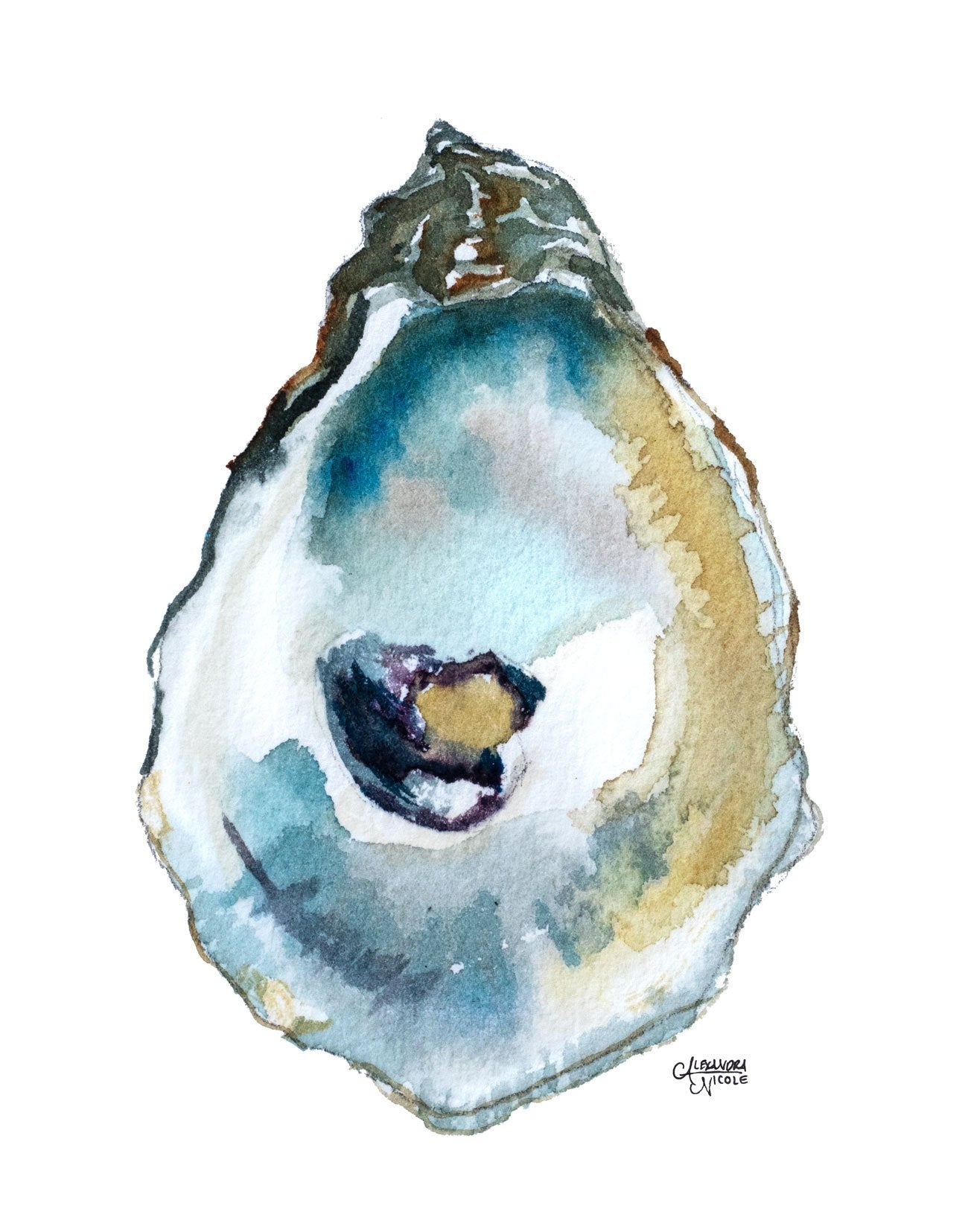The image is a handmade watercolor painting of an oyster shell centered against a plain white backdrop. The shell is depicted vertically, with its pointy end towards the top and its rounder end at the bottom. The exterior of the shell features shades of gray and brown, mimicking the natural, rugged texture of an oyster. The interior brims with a palette of vivid colors: dark and light blues dominate the top and bottom, gracefully flowing into gold and pale yellow hues along the right-hand side. The shell's curvature is accentuated by undulating lines that convey its three-dimensional form.

At the heart of the oyster, there's a focal point—a dark swash of watercolor encircling a golden orb, likely representing a pearl, nestled within the vibrant blue and teal pigments. The sandy textures within the shell add depth and realism, enhancing the tactile quality of the painting. 

At the bottom of the painting, in elegant black handwriting, is the artist's signature, "Alexandra Nicole," giving the piece personal authenticity. The overall composition beautifully captures the delicate yet intricate nature of an opened oyster shell.